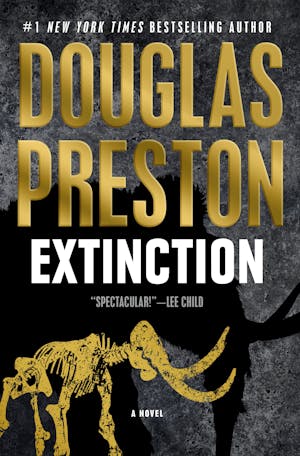The captivating book cover of "Extinction," a novel by Douglas Preston, features a grey textured backdrop that mimics stone. Prominently displayed at the top in white lettering is the accolade "Number One New York Times Best Selling Author." The author's name, Douglas Preston, is emblazoned in large gold letters, immediately catching the eye. Below, the book title "Extinction" stands out in bold white text. A notable quote from Lee Child, “Spectacular,” is showcased beneath the title in smaller white lettering. Towards the bottom left of the cover, there is a detailed gold depiction of what appears to be a dinosaur or fossilized tusks, with a larger black shadow looming behind it, adding a sense of depth and mystery. Just beneath the fossil's head, in small white letters, the word "Novel" subtly indicates the book's genre.